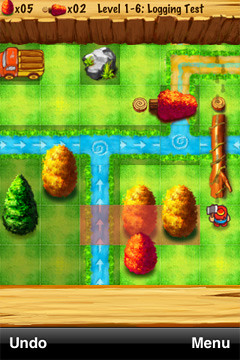This still image, taken from a video game, presents a bird’s-eye view of a lush landscape marked by vast green grass fields. A winding water canal, complete with directional arrows, traverses the scene from the bottom edge of the frame across its entire width. Within the verdant fields, detailed icons symbolize various elements: a prominent rock icon, an old, weathered pickup truck, and a collection of trees. A notable feature is a fallen log stretching across the water, serving as a makeshift bridge. Approaching this log is the player’s small, animated game character brandishing an axe, seemingly ready to interact with the environment.